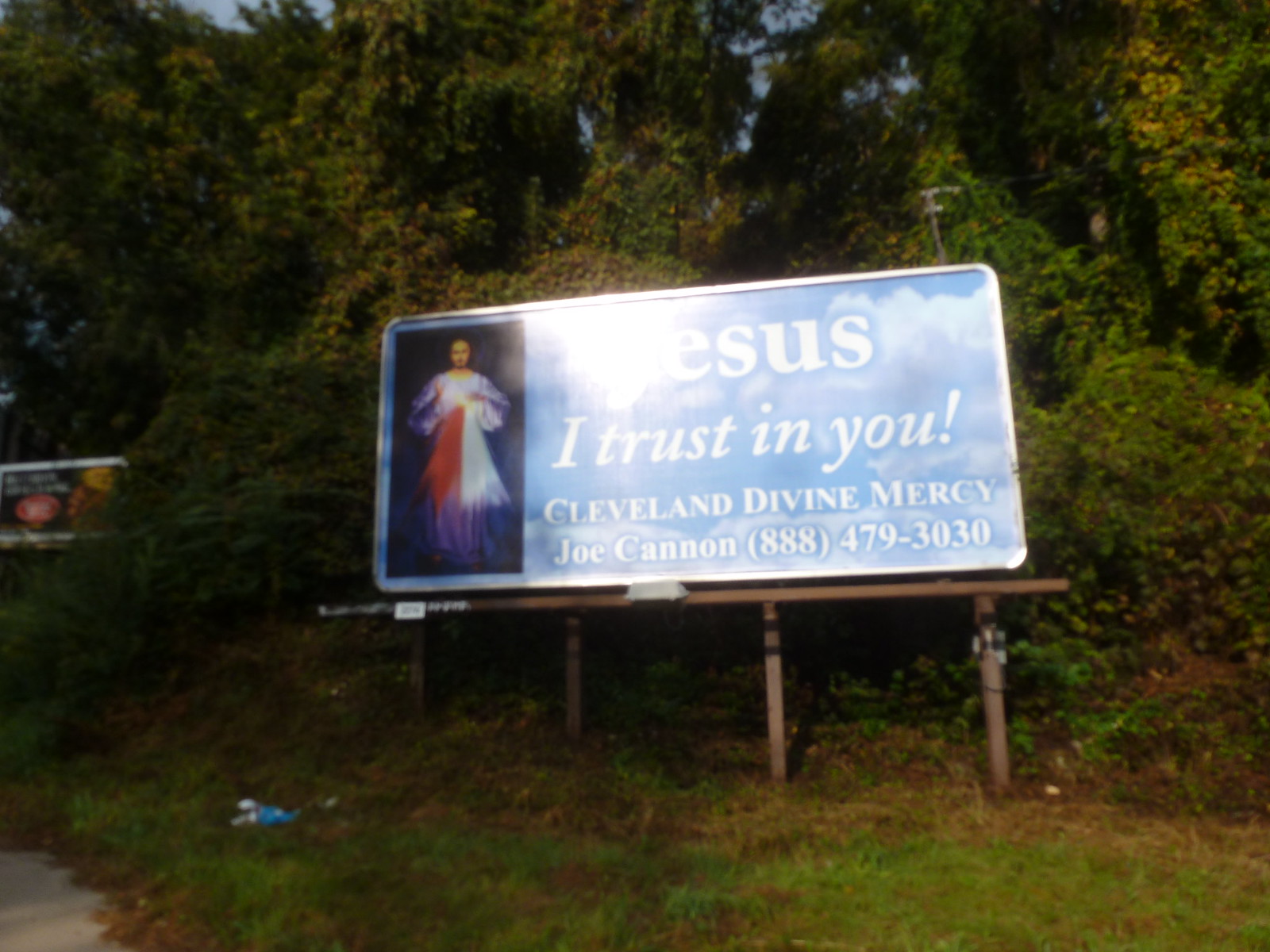Caption: 

An eye-catching full-size billboard stands prominently on the side of a busy road, mounted securely on a horizontal frame supported by four vertical posts. The billboard features smooth, curved edges that create a modern, polished appearance. Captured in the photograph is a reflection created by the sun, adding a striking highlight to the advertisement's surface.

The main visual on the left side of the billboard depicts an ethereal image of Jesus Christ, adorned in a long, flowing gown with a shawl elegantly draped over one shoulder. Accompanying this serene imagery, the text reads: "Jesus, I trust in you, Cleveland Divine Mercy, Joe Cannon, 888-479-3030," set against a peaceful blue sky filled with soft, billowing clouds.

Encompassing the scene is a backdrop of dense foliage, with trees, bushes, and shrubs forming a natural border. Notably, a minor distraction is present in the lower left corner of the image, where a few pieces of litter are visible, contrasting with the otherwise tranquil setting.